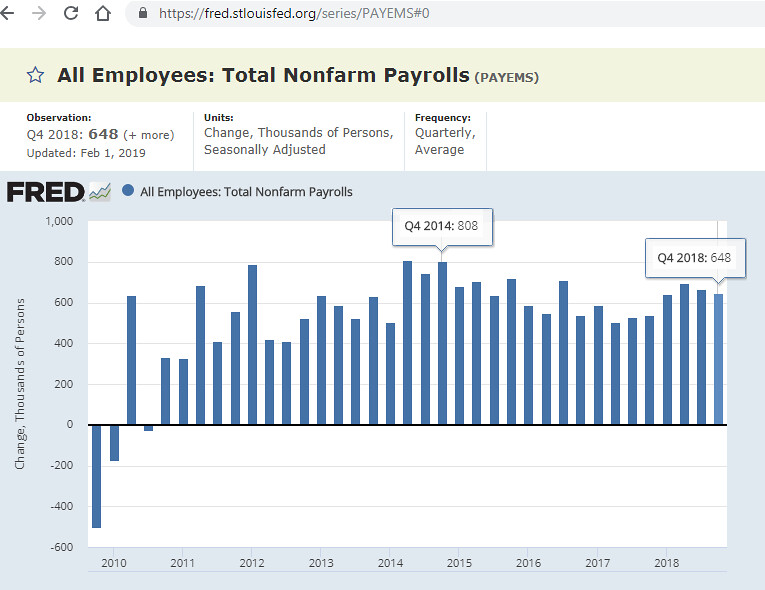The image is a digital screenshot of a bar graph from a website displaying data titled "All Employees: Total Non-Farm Payrolls." This chart, sourced from FRED, shows the fluctuation of payrolls over several years, specifically from 2010 to 2018, with an update as of February 1, 2019. It includes various descriptive metrics such as "Observation: Q4 2018," which marked a payroll change of 648, "Units: Change in Thousands of Persons (Seasonally Adjusted)," and "Frequency: Quarterly Average." The chart is depicted with bars in blue, representing payroll changes in thousands of persons each quarter. Notably, the highest payroll change was 808 in Q4 2014, while the lowest was around -500 in 2010. The colors involved in the image include green, black, white, blue, and orange.